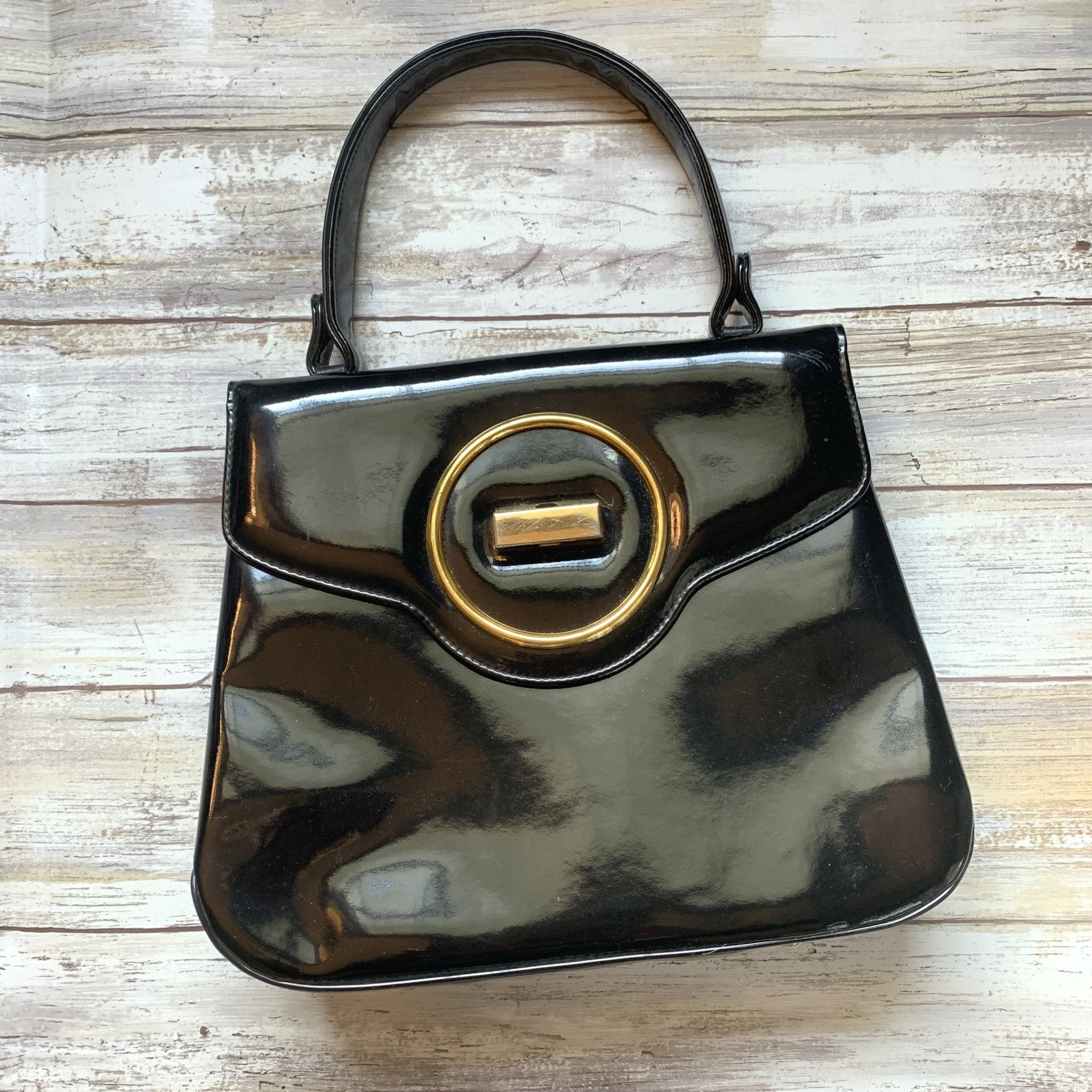The image features a photograph of an elegant, high-end black purse made from shiny, rigid material, likely vinyl or leather. The purse is rectangular with slightly rounded bottom edges, giving it a trapezoidal shape. It has a single black strap, suggesting it is designed to be carried by hand or at the elbow rather than worn cross-body or over the shoulder. The closure consists of a triangular flap adorned with a striking gold circle, which has a rectangular mechanism in the center that likely serves as a latch. The purse is laid on a weathered wooden deck with multiple grayish-white panels that form the background, adding a rustic contrast to the sleek, sophisticated look of the purse. The purse is tilted slightly to the left in the photo, highlighting its refined craftsmanship and luxurious appearance.